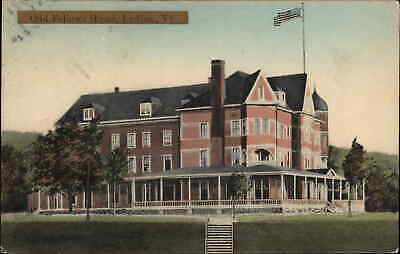The image depicts a large, mansion-like building constructed from red brick. This expansive structure is adorned with numerous windows and a distinctive wraparound porch, providing an extensive view of the surroundings. The building features many peaks and a central widow's peak, from which an American flag is flown. The roof is covered in black tar and includes a chimney at the fore end. The mansion is situated on a vast, square-looking hill with a manicured lawn, where white concrete stairs descend to a lower level, adding to the grandeur. Surrounding the structure, there are several trees, both behind and adjacent, with a pale, whitewashed sky in the background, contributing to the historic and stately ambiance of the scene. The overall palette of the image includes dark, muted colors with a combination of red, black, white, and shades of green from the lawn.